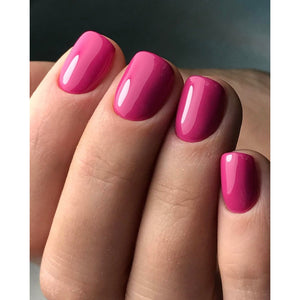In this close-up color photograph, the focal point is a woman's upturned palm with her fingernails prominently displayed. The image captures the fingertips of her index finger at the upper left, progressing diagonally towards her pinky finger near the bottom center right, showcasing four well-groomed, short-trimmed nails painted with glossy dark pink polish that reflects light, indicating the light source is positioned to the left. The nails’ shine creates a bright, almost white highlight on the left side of each nail. The woman’s tan skin tones display a light beige hue with a hint of pink, while the background above her hand features a dark gray, slate-blue gradient. The thumb is barely visible on the left side, tucked behind the index finger, and a portion of her palm is shown in the middle right background of the image. The photograph’s style is detailed and realistic, emphasizing the smooth texture and reflective quality of the nail polish against the soft, shaded contours of her fingers and palm.